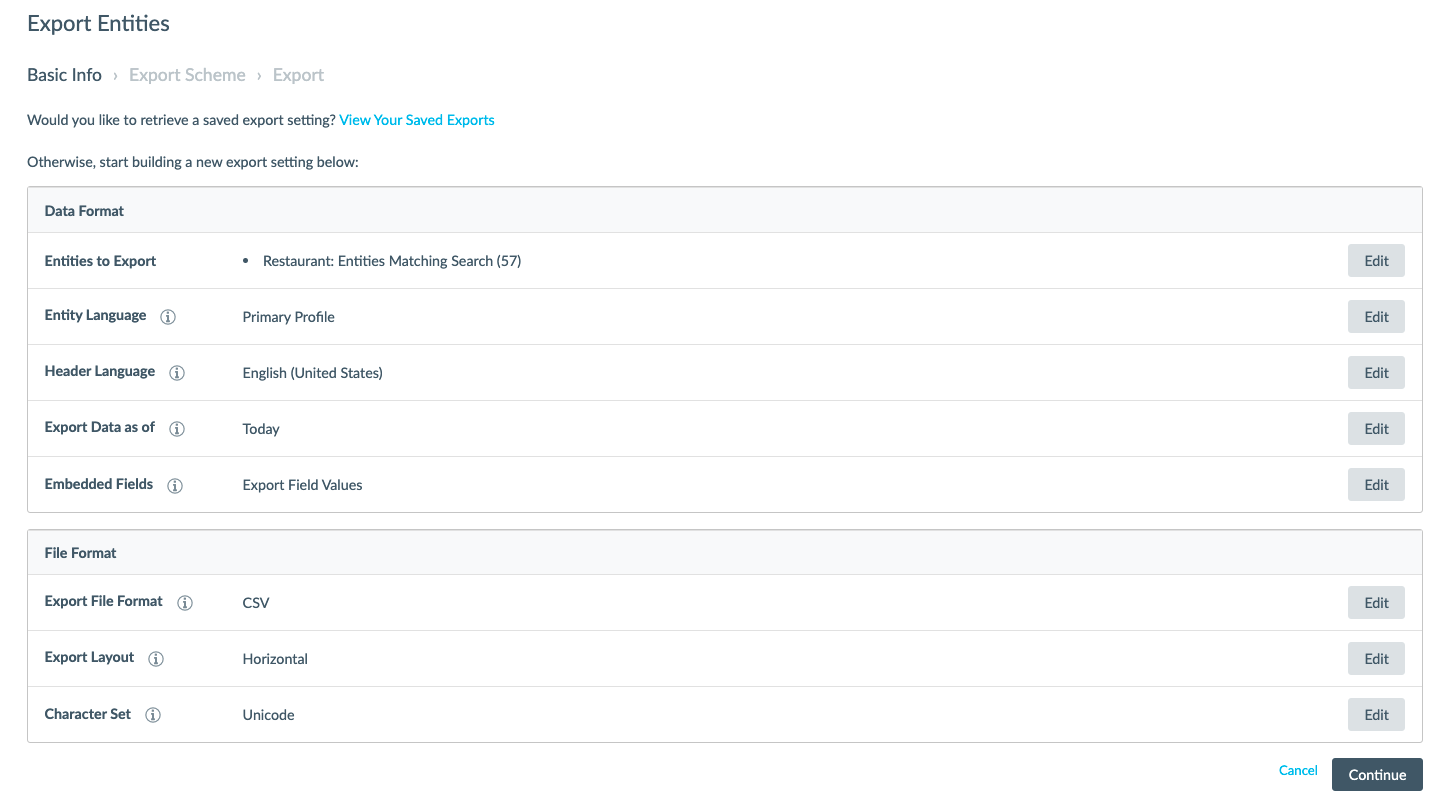**Detailed Descriptive Caption:**

The image depicts a screen from a business software interface designed for exporting data. At the top, there are labels indicating different sections such as "Export Entities," "Basic Info," "Export Scheme," and "Export." A prompt asks the user if they would like to retrieve saved export settings or view saved exports, highlighted in blue. The alternative option provided is to start building a new export setting below.

The interface is organized into several categories with the following settings and options:
1. **Entities to Export:** This category shows "Restaurants" as the currently selected entities, with 57 matching entries, and includes an "Edit" button.
2. **Entity Language:** Designated as "Primary Profile" with an exclamation mark for attention.
3. **Header Language:** Set to "English, United States."
4. **Export Data As Of:** Specified as "Today."
5. **Embedded Fields:** Set to "Export field values."

Following these, there's a section titled **File Format** with the following options:
1. **Export File Format:** Set to "CSV."
2. **Export Layout:** Configured to "Horizontal."
3. **Character Set:** Set to "Unicode."

At the bottom right of the interface, there are two buttons – a blue "Cancel" button and a "Continue" button. The overall design features a traditional white background with standard plain blackish text, creating a straightforward and user-friendly appearance. This export settings interface appears to offer detailed customization options, though the exact purpose of the software remains unidentified.